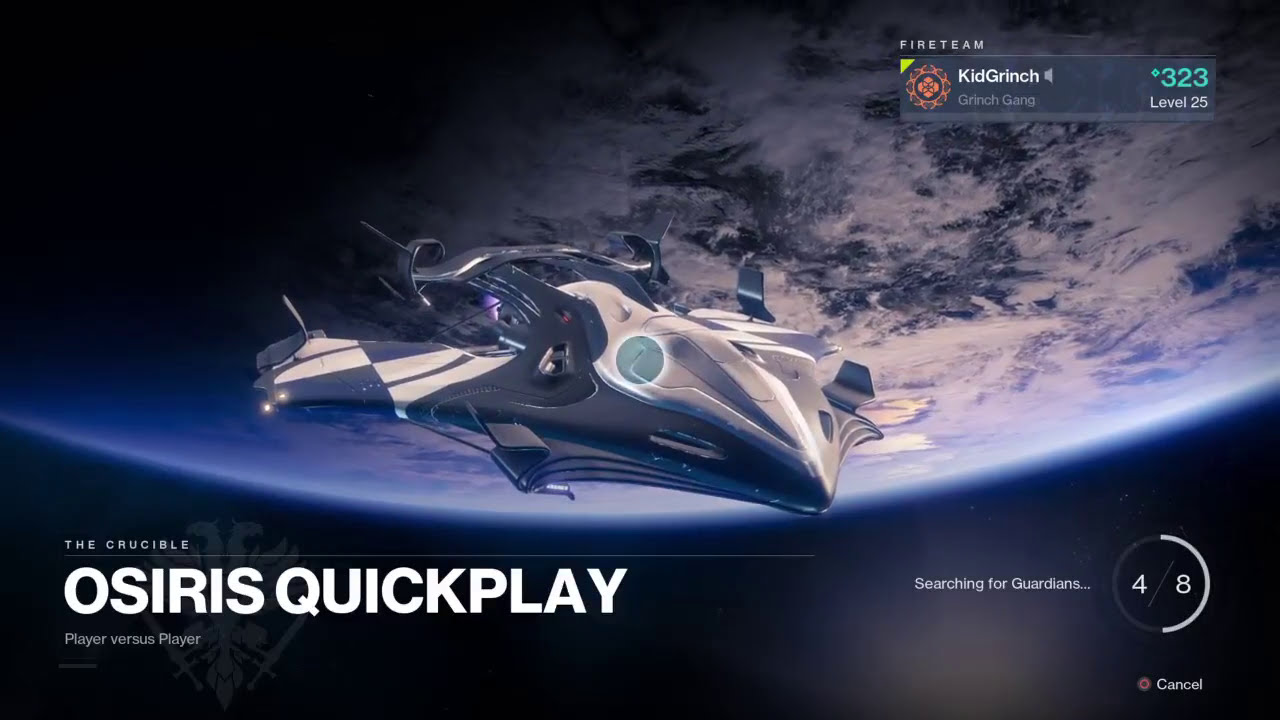The image is a colored digital screenshot or promotional poster for a video game titled *"The Crucible: Osiris Quick Play"*, a player versus player game. Dominating the center of the image is a white and gray futuristic spacecraft set against the backdrop of a large planet with a thick atmosphere of white clouds, indicating a celestial, space-themed environment. Below the spacecraft, a vast expanse of black space stretches out. The bottom left corner of the image displays the game's title in large white capital letters: "THE CRUCIBLE: OSIRIS QUICK PLAY". In the bottom right corner, it states "Searching for Guardians" with a half-completed circle showing "4/8" inside it, and below that, the word "Cancel" is written. In the top right corner, there is a rectangular gray box featuring a logo on the left, followed by "Kid Grinch, Grinch Gang, Degree 323, Level 25". Above this box, the text "Fire Team" is displayed. The overall composition creates a vivid impression of an intense, space-based multiplayer game.